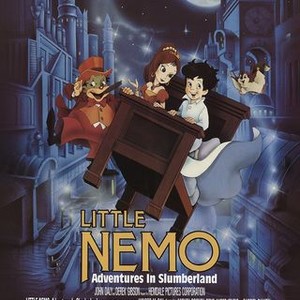This image is a highly detailed movie poster, possibly also serving as a book cover, for the children's story "Little Nemo: Adventures in Slumberland." The title "Little Nemo" is prominently displayed at the bottom in large gold letters with a black outline, while the subtitle "Adventures in Slumberland" appears below it in smaller white text, with hard-to-read white writing further down. The scene is set at night, as illustrated by a dark sky filled with stars and a partial moon in the upper right corner. Flanking the scene are bluish-gray buildings on both sides, adding to the nighttime cityscape ambiance. At the center of the image, Little Nemo, a young boy in a white collared shirt, and a girl in a red princess outfit with flowing brown hair, are joyfully flying through the city sky on a brown wooden bed with a white mattress and blanket billowing behind them. Accompanying them is a whimsical character, a frog man in a red suit and top hat, situated to their left. There's also a small, cheerful flying squirrel to the upper right of the bed. Swirls of sparkles surround them, enhancing the magical feel of their night-time adventure. The overall image is vibrant and festive, capturing the lively and fantastical essence of Little Nemo's journey through Slumberland.